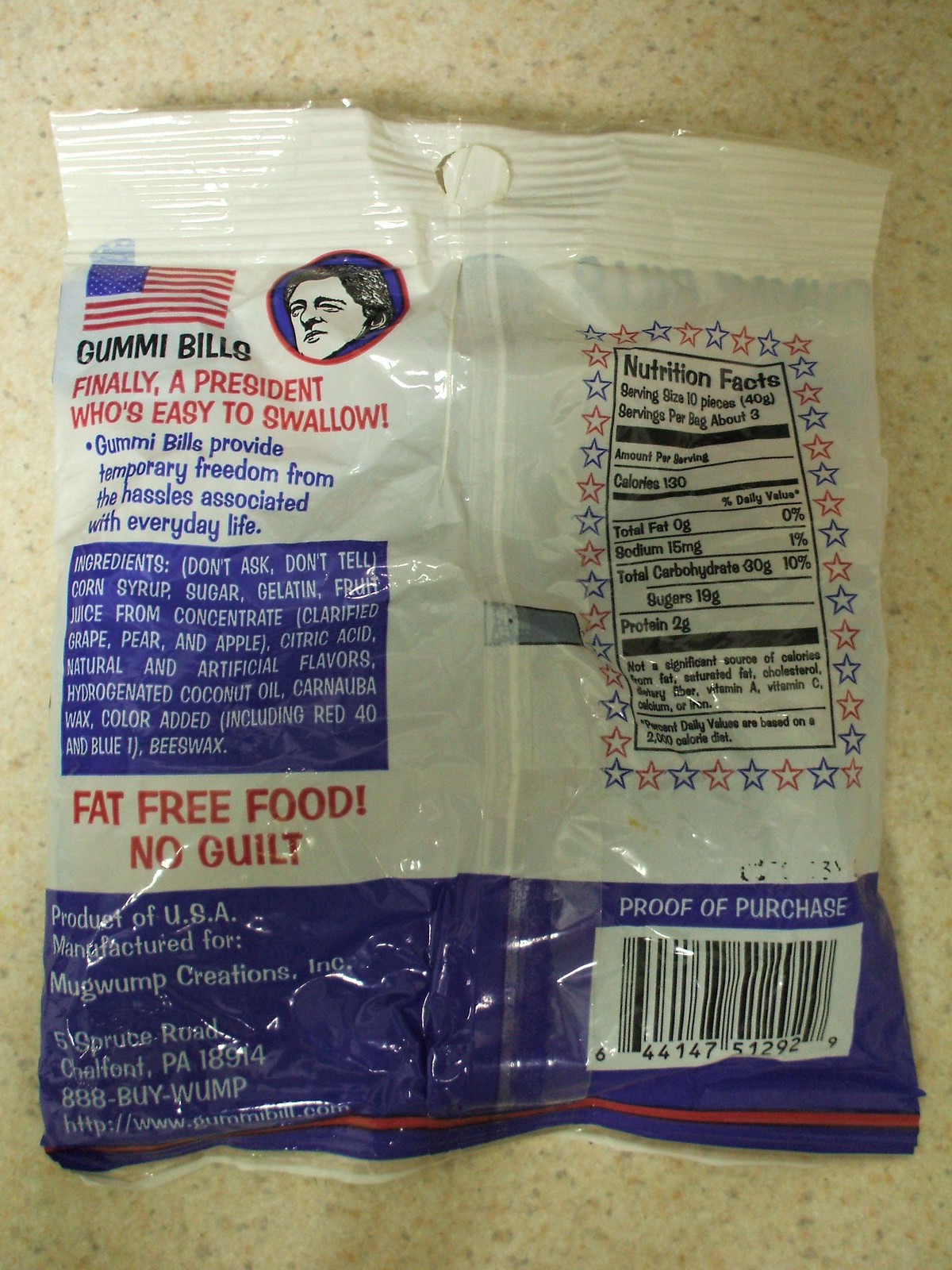This image features the back side of a plastic packaging for a snack. On the left side of the bag, there is a prominent Nutrition Facts chart, bordered by stars with alternating red and blue outlines. The right side of the bag showcases a small flag at the top, followed by a cartoon image. Beneath the cartoon, the text reads, "Gummy Bills: Finally, a president who's easy to swallow." Below this slogan, an ingredients box with a blue background details the snack's contents across approximately six lines of text. Highlighted in bold red text is the phrase, "Fat-free food, no guilt." The bottom section of the bag has a blue border displaying the manufacturer's name, the country of origin ("Product of the United States"), and the address. On the right side of this border, there is a proof of purchase area along with a barcode.